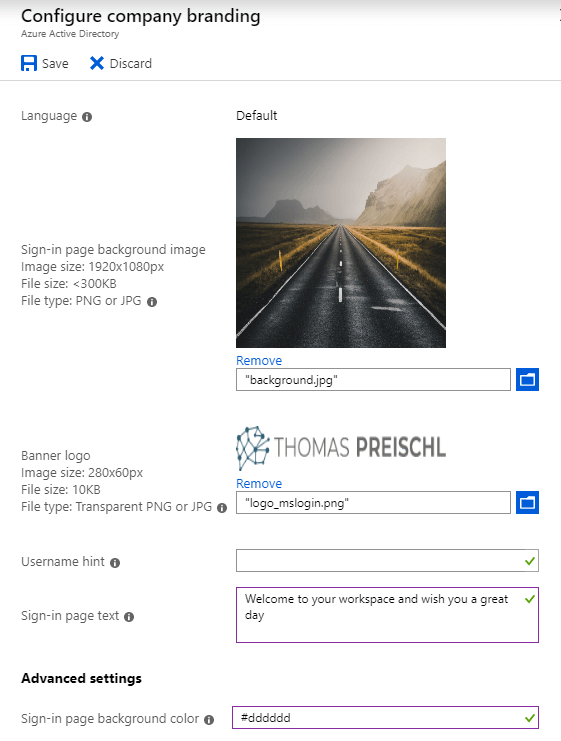Sure, here's a cleaned-up and detailed caption for the image:

---

Detailed Caption: Screenshot of an Azure Active Directory customization interface. The interface is set against a clean white background and prominently features a sample image of a long, straight road cutting through a barren, desert-like landscape with dry mountains in the distance. The image customization program offers various editable fields and settings organized neatly on the screen.

Key elements include:

1. **Header and Banner Section**: Options to upload files, including the main image and a logo or banner.
2. **Text and Language Settings**: Fields to input and overlay text onto the image, with the ability to choose the text color, font, and size. The text displayed appears in a dark gray hue.
3. **Username Input Field**: A space designated for entering usernames, perhaps for sign-in or personalization purposes.
4. **Advanced Settings**: Offers features such as selecting the background color for the sign-in page, with input fields for specific color codes.
5. **Save and Discard Buttons**: Clearly labeled buttons to either save the changes made or discard them.

This interface appears to function as a basic editor, potentially for creating custom sign-in pages or backgrounds for web applications, providing a straightforward and user-friendly experience.